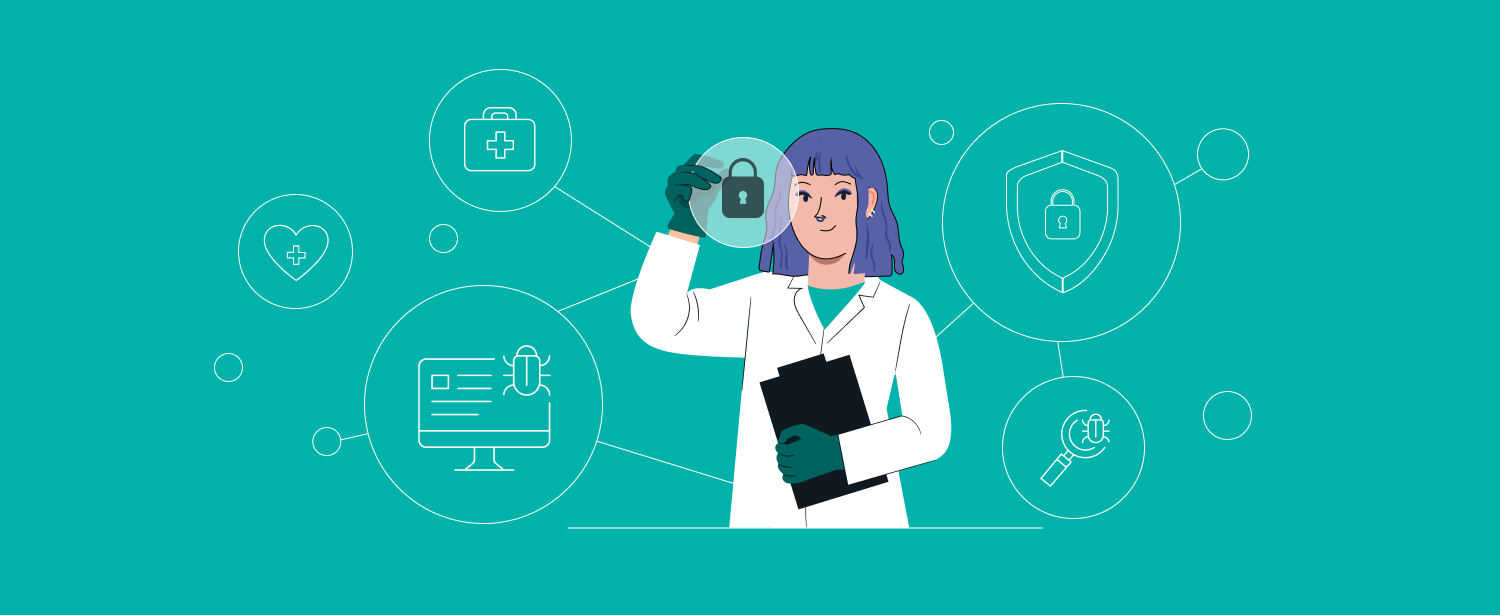The image is a detailed cartoon illustration set indoors, depicting a female doctor or lab assistant with light skin, possibly of Asian or white ethnicity. She has purple hair that reaches her neck and is smiling at the camera. She wears a white lab coat over layered yellow and green shirts, coupled with green gloves. In her left hand, she clutches a black clipboard, while her right hand holds a padlock. The background of the image is green, adorned with a series of interconnected white lines and circular graphics. To the left, there is an upward arrow leading to a circle enclosing a first aid kit, beneath which is a computer monitor displaying a bug. To the center-left is a circle with a heart symbol, while to the center-right there is a shield with a padlock, likely symbolizing cybersecurity. Further below, a circle encloses a magnifying glass and a bug, potentially indicating antivirus or research work. The image is bright, clear, and highly detailed with no text present, possibly designed for a website or informational graphic.